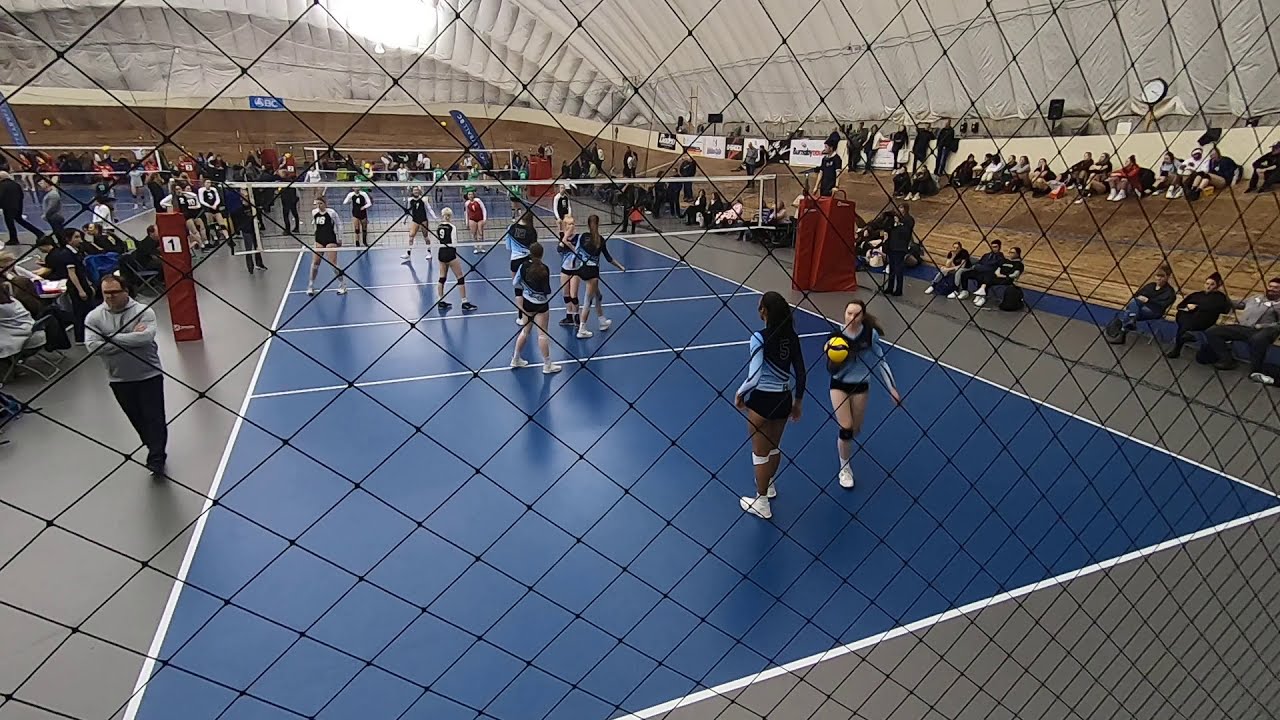In this detailed indoor scene of a volleyball competition, girls are actively playing on multiple blue courts, each bordered with white lines. The entire event is held inside a dome-like, inflatable arena with white, air-filled walls and ceiling. The main court in the foreground features teams of girls in light blue long-sleeved shirts, black shorts, and white shoes competing against teams in black uniforms. One girl is notably holding a yellow volleyball. Surrounding the courts, gray floors extend outwards, with spectators seated on wooden planks and brown bleachers. There are several courts visible, including one prominently in the upper left-hand side of the image. Red foam padding secures the poles holding the volleyball nets. A referee stands elevated on a red podium to oversee the match, all under the watchful eyes of numerous spectators filling the venue.